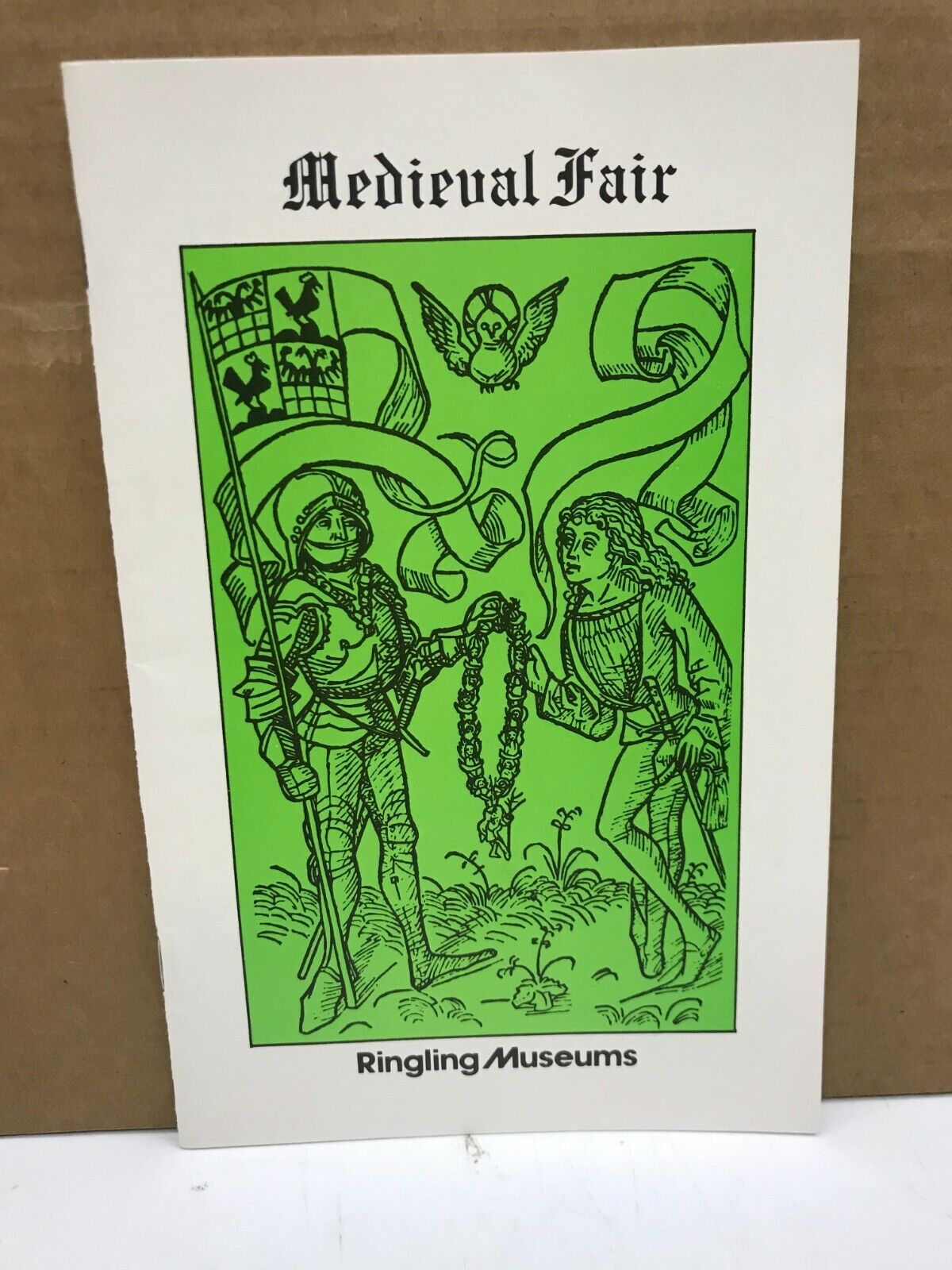This image features an advertisement, possibly a flyer or a poster, with a detailed illustration. The white paper displays "Medieval Fair" prominently in black text at the top. Below this title, an intricate illustration occupies a green background with black ink detailing. The artwork depicts a medieval scene: a knight in full armor, helmeted, holding a large flag, and with a sword near his leg. Beside him stands another figure with long curly hair, dressed in regular medieval attire, who also has a sword by their hip. The figures appear to be exchanging or holding a wreath. A bird is illustrated flying in the sky above them. At the bottom of the advertisement, it reads "Ringling Museums" in black text. The paper is resting on a white surface with a brown background behind it.